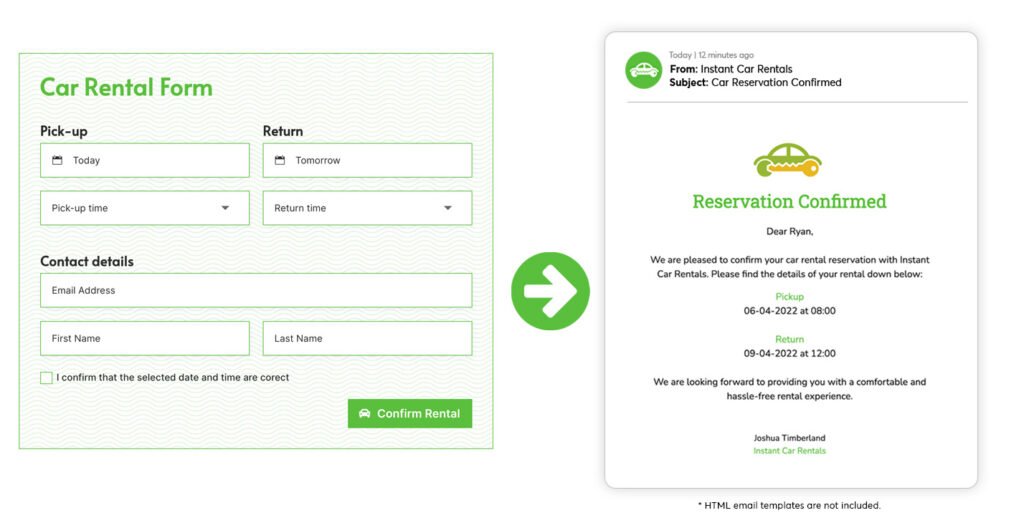The image features a detailed car rental form within a gray box, prominently displaying various fields and details in green text. At the top, "Car Rental Form" is marked in green. Beneath it, there are sections for "Pickup" and "Return". Under the "Pickup" section, the date is set to "Today", and under the "Return" section, the date is listed as "Tomorrow". Both sections include specific times for pickup and return.

The form continues to request "Contact Details", featuring input boxes for "Email Address", "First Name", and "Last Name". Below these fields, an unchecked checkbox is labeled "I confirm that the selected date and time are correct".

At the bottom of the form, a green rectangle button with white text reads "Confirm Rental". Next to this button, a notification in green text announces "Reservation Confirmed".

Adjacent to this form, there is an image of a green car accompanied by a yellow key. Above the image, a message addresses "Dear Ryan", informing him of the confirmation of his car rental reservation through Instant Car Rentals, with details listed below. The pickup time is specified as 06-04-2022 at 8:00 AM and the return time as 06-05-2022 at 12:00 PM. The message eagerly looks forward to providing a comfortable and hassle-free rental experience. 

The signature at the end reads "Joshua Timberland" from Instant Car Rentals, highlighted in green. Below this, there is a note marked with a star, stating "HTML email templates are not included".